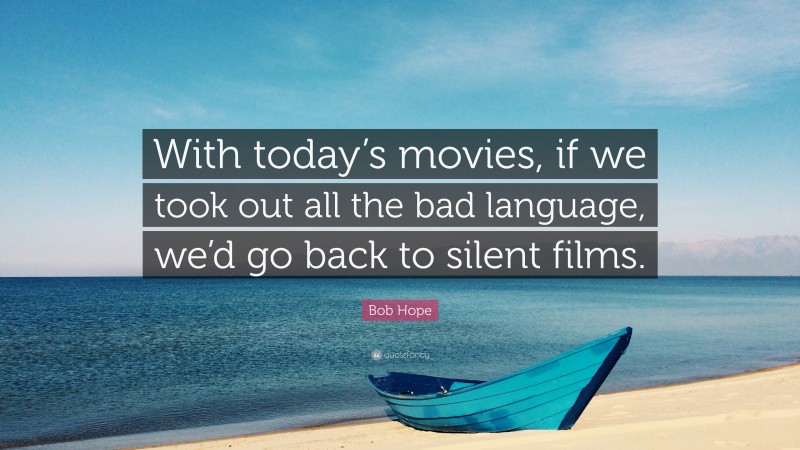The image is a photograph featuring a serene beach with pristine white sand and a small, vivid blue rowboat resting on the shore, right next to the calm, clean blue waters of the ocean. In the distance, a volcanic island—possibly part of Hawaii—adds to the scenic beauty beneath a clear blue sky dotted with a few white clouds. Overlaid in the center of the image is an inspirational quote in bold white letters on a black background that reads, "With today's movies, if we took out all the bad language, we'd go back to silent films." The quote is attributed to Bob Hope, with his name appearing in smaller white letters against a purple-pink background below the text.